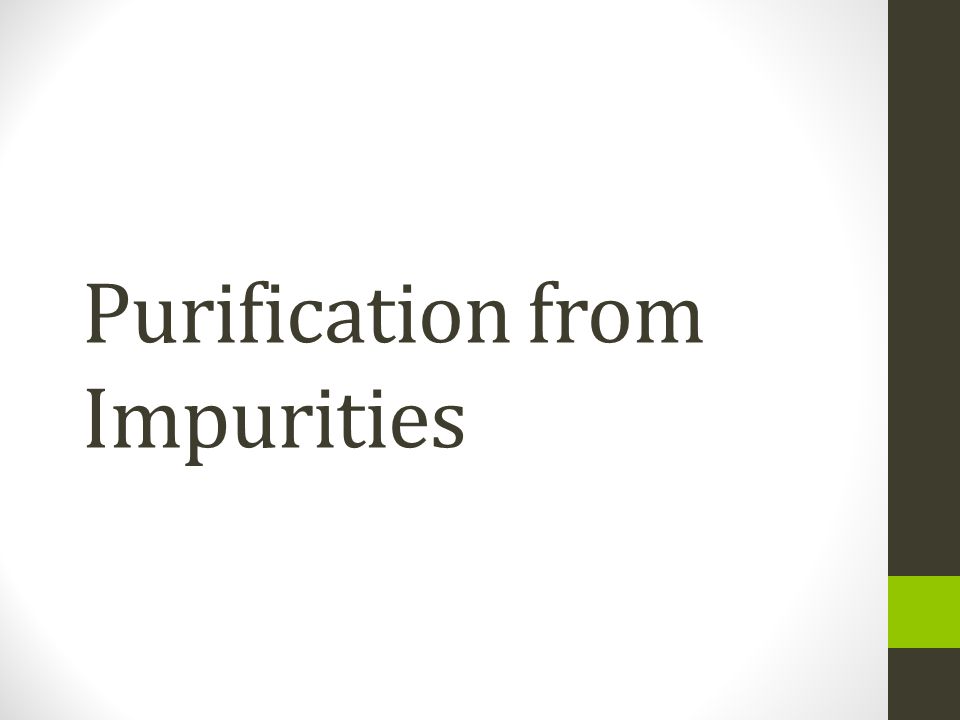This digitally synthesized image, likely a PowerPoint slide for a science presentation, features a minimalist design with a white background accented by dark gray gradients in the top left and bottom left corners. Dominating the right side is a vertical dark gray column that extends from the top to the bottom of the image. Near the lower portion of this column is a small lime green square that partially obscures the gray area. Large black text centered in the middle of the image reads "purification from impurities," with "impurities" aligned beneath and toward the left, using the same font style and color. The overall design is clean and uncluttered, with no additional objects or people, emphasizing the textual content.